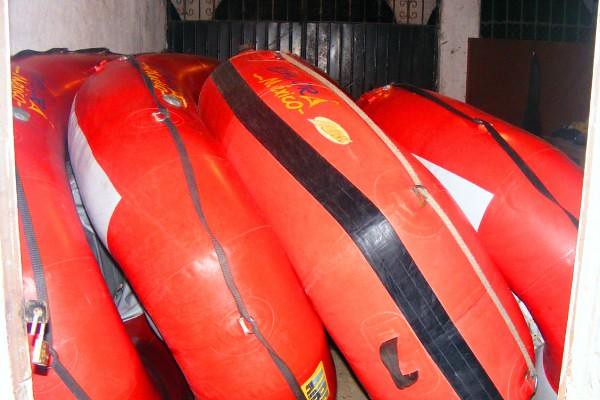This horizontal rectangular color photograph captures a cluster of four large, red inflatable rafts arranged on their sides, leaning against each other and facing a black ironwork gate on the right side of the frame. Each raft features a prominent yellow "Mexico" inscription and a thin black stripe encircling its center, adding to their uniform appearance. Some rafts have visible handles and ropes along their edges, suggesting their use in water-based tourist activities. The background reveals part of a white wall and a black metal structure, which resembles a patio area with metal fencing or grating. The rafts partially appear cut off at the edges of the photograph, enhancing the sense of a crowded storage area. The scene is brightly lit with artificial light, emphasizing the glossy texture of the rafts. There are no people, animals, plants, flowers, trees, or motorized vehicles present in this image.